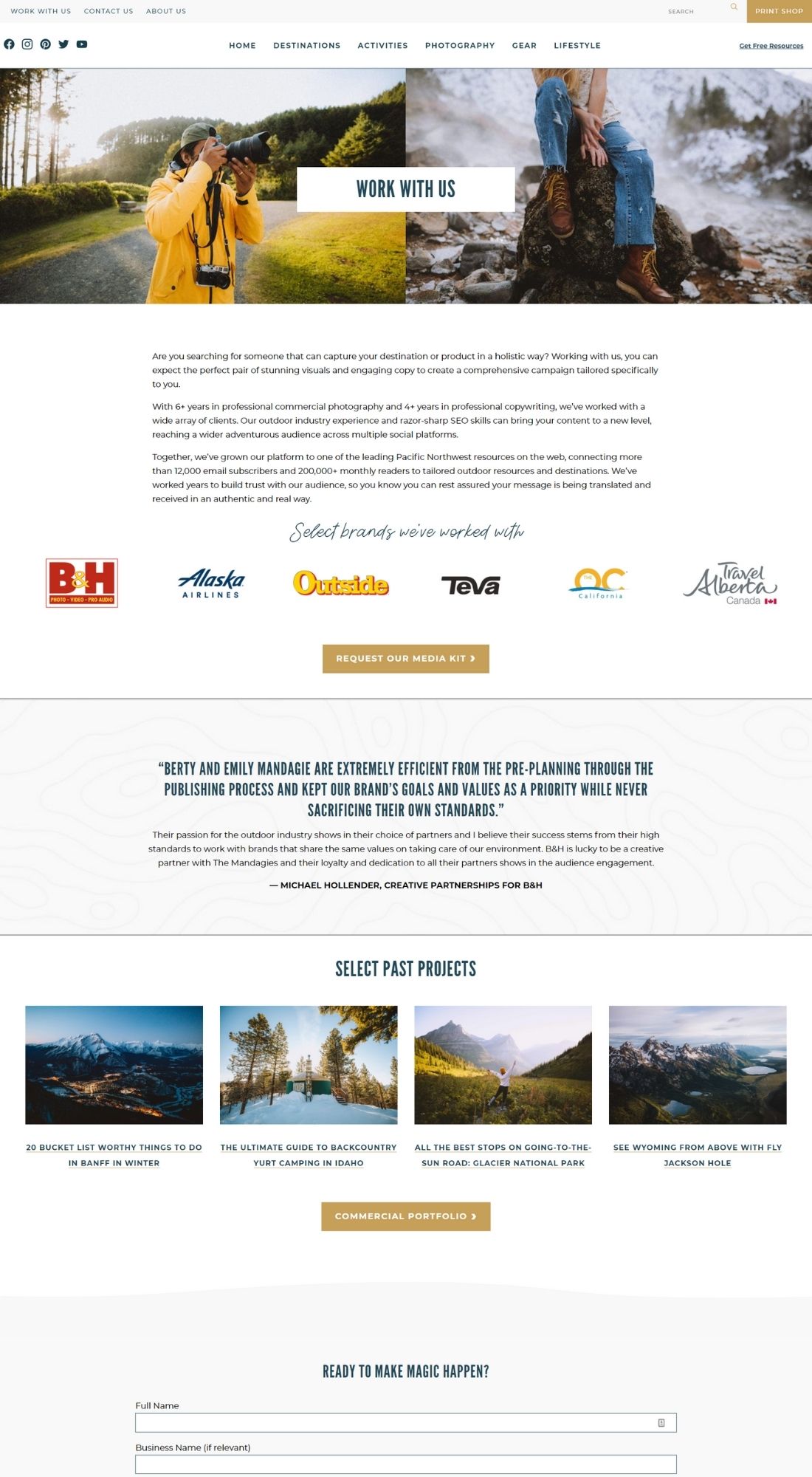The screenshot captures a meticulously designed homepage of a photography-based website. 

At the very top left, the navigation menu features options for "Work With Us," "Contact Us," and "About Us." Adjacent to this, on the top right, the menu includes a "Print Shop" link, with a conveniently placed search bar immediately to its left. Below this primary navigation, a secondary menu in the top middle displays categories in sequence from left to right: "Home," "Destination," "Activities," "Photography," "Gear," and "Lifestyle." Additionally, on the far left of this menu, there are social media icons linking to Facebook, Instagram, Pinterest, Twitter, and YouTube, while the far right features a link labeled "Gift Resource."

Centered beneath these navigation elements, the layout transitions into a visual split. On the left, a rectangular image features the text "Work With Us" superimposed on a captivating scene of a person taking a photograph on a road that meanders through a lush wilderness. The right side displays another rectangular image, this time showing a woman seated on a rock, evocative of adventure or exploration.

The middle section of the page prominently showcases logos of several prestigious brands that the website collaborates with, including "H," "Alaska Airlines," "Outside," "Viva," "OC California," and "Travel Alberta." Below these logos, in a clearly defined box, visitors are invited to "Request Our Media Kit," encouraging further engagement.

Overall, the page is both visually appealing and intuitively organized, catering seamlessly to photography enthusiasts and potential collaborators.